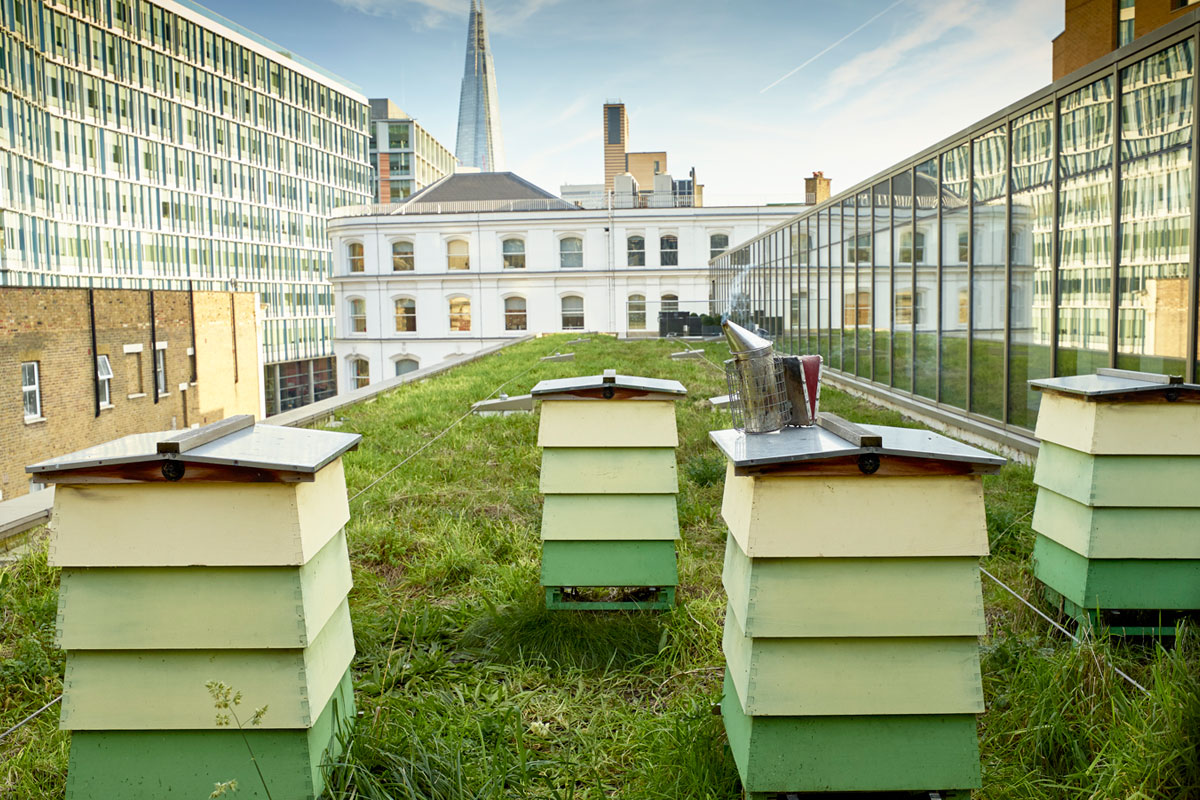In this unusual urban scene, a rooftop covered in grass serves as the setting for four distinct beehives. The hives are painted in a gradient of colors, with the bottom slat in a vibrant dark green, transitioning to a pale green, and topped with a light yellowish hue. Each hive is built in a shingled, clapboard style with barely slanted roofs. On one of the hives, there is beekeeping equipment, including a smoker and a mesh container, tools essential for collecting honey.

Surrounding this green oasis, a juxtaposition of modern architecture and older buildings frames the view. To the right, a glass-walled building reflects the cityscape, while to the left, a massive structure with six rows of windows above its two-story base looms large. Beyond the beehives, a white building with a steeple-like top towers above, featuring multiple rows of windows that give it a church-like appearance. This intriguing mix of natural and urban elements invites exploration and adds a unique character to the city skyline.